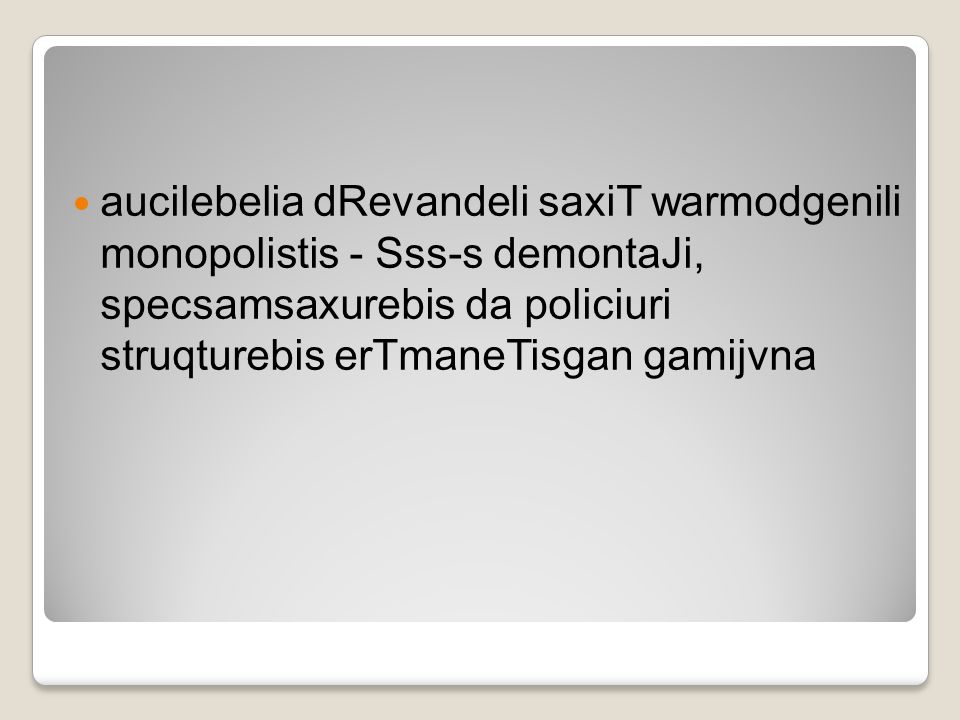The image depicts a PowerPoint-style presentation slide with a two-toned gray background, transitioning from a lighter gray in the middle to a darker gray towards the edges and corners. The slide is framed by a thin white border, which is itself encased in a light tan or beige outer border. Dominating the center of the slide is a piece of text written in black and punctuated by a single bright orange bullet point. The text appears to be in an indiscernible, possibly fabricated, language, featuring terms like "Oscillabilia D. Rivandelli Saxi T. Wormaud Genelli Monopolists S. S. S. S. D. Montagee Spexam Saxe Erebus Da Politicuri Structuribus Ertemain Tiscon Gamivana." This arrangement, with no discernible meaning and a mismatch of capitalized and lowercase letters, suggests that the text may be gibberish rather than an actual language. The overall impression is that of a deliberately styled, formal presentation slide, carefully segmented by its various shades and borders.